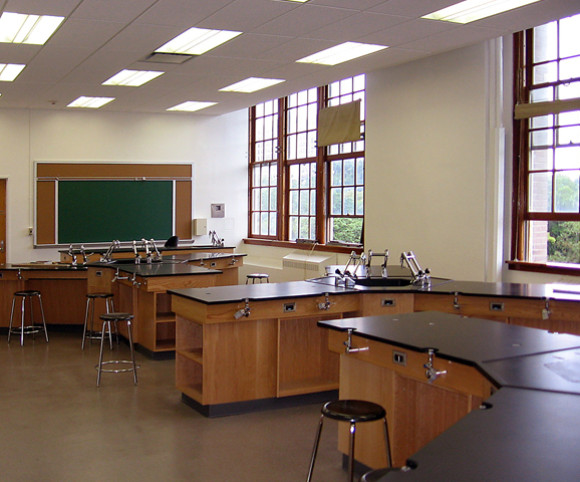This color photograph depicts an unoccupied classroom that appears to be designed for science activities, possibly a biology or chemistry lab. The room features several long tables with black tabletops and integrated wooden storage spaces beneath, accompanied by black and silver stools. Dominating one wall is a large green chalkboard with the words "Nothing Road" written on it. The classroom is highly illuminated by natural light streaming in through four enormous windows, of which two are open to allow fresh air inside. Beneath one windowsill resides a white wall heater. The vibrant daylight outside reveals a view of a lush forest, indicating the classroom is situated on an upper story, likely the second or third floor. Additionally, there are two sinks that might serve as washing stations, hinting at the laboratory function of the room. The lights on the ceiling are switched on, adding to the room's bright and inviting ambiance.